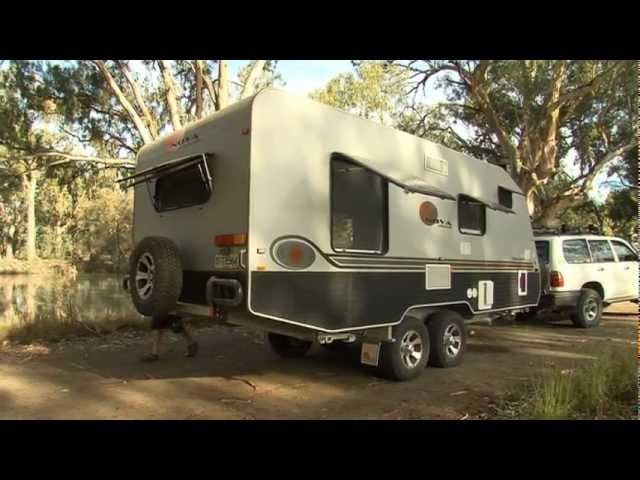The outdoor color photograph captures a serene camping scene dominated by a white travel trailer accented with brown along its lower quarter. The trailer, labeled "Nova," is approximately 15 feet long and features a sleek, clean exterior with no visible dirt or damage, suggesting it’s brand new. The trailer has three side windows and one rear window, all propped open at about a 45-degree angle, enhancing the inviting camping atmosphere. A spare tire is attached to the back, and there are utility outlets at the lower front portion. The trailer is being towed by a white station wagon, discernible by its position and connection, though partially out of frame.

The setting is a picturesque campground that appears to be in California, identifiable by the types of trees in the background, hinting at a summer or springtime ambience. The vehicle and trailer are parked on a dirt road beside a tranquil pond, whose surface softly reflects the surrounding greenery. Trees and lush foliage create a natural backdrop of shade and tranquility. A child's legs are visible behind the trailer, adding a touch of human presence without distracting from the tranquil environment. This photograph, lit by natural light, captures the idyllic essence of a camping getaway.